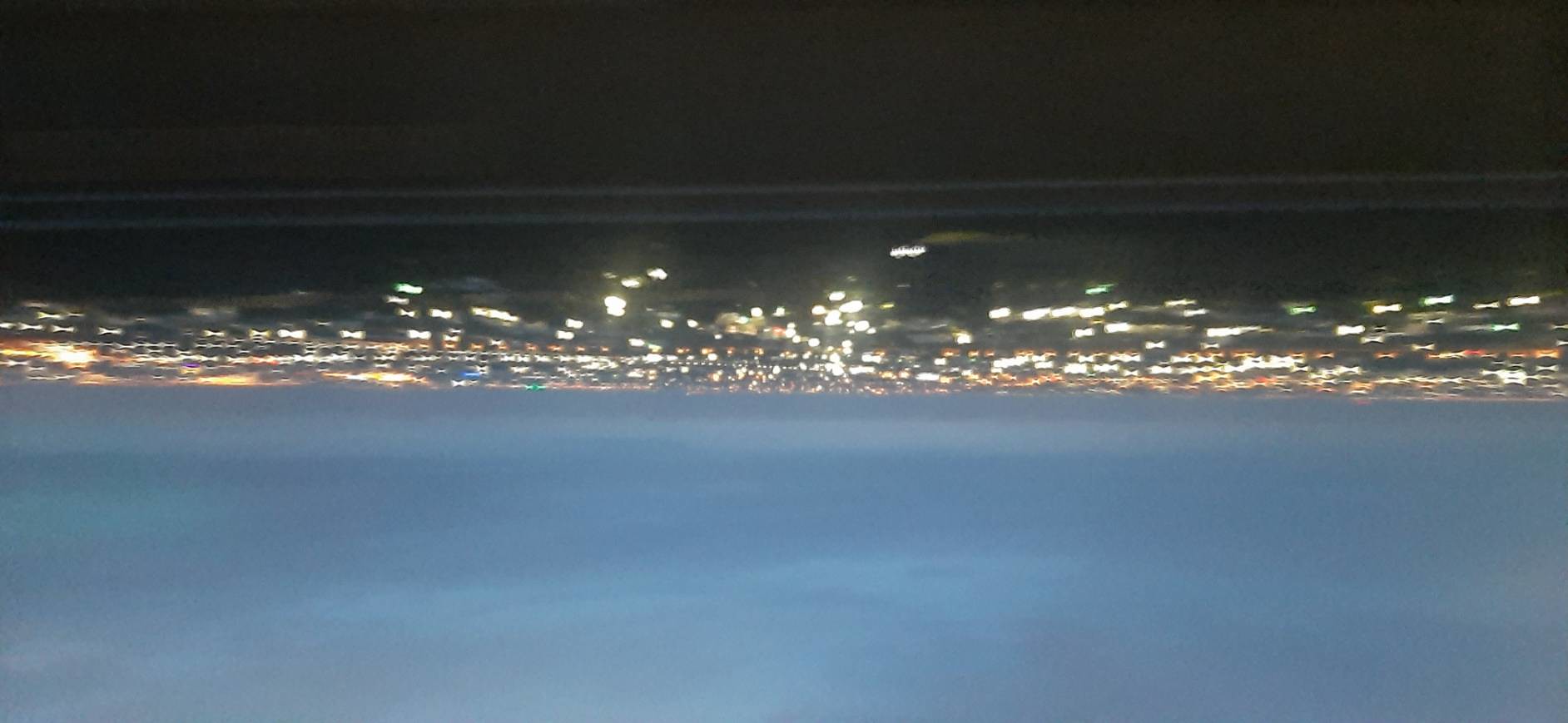This color photograph, although blurry and dark, presents a captivating and somewhat puzzling scene. At first glance, it appears to be an upside-down cityscape captured at dusk. The upper portion of the image is enveloped in darkness, punctuated by two thin grey lines that run horizontally, resembling a road. Beneath this, an array of blurred lights stretches across the width of the photograph, evoking the appearance of city lights or car headlights seen from above. These lights give the impression of vibrant activity amidst the obscurity. Towards the bottom, a bluish expanse suggests the presence of the sky, interspersed with greyish clouds, creating a diffused mix of blue and grey hues. This lower section subtly mirrors a seascape or even a mountainscape, adding to the image's ambiguity. However, considering the indicative road, the scene most plausibly represents an inverted photograph of a city at dusk.